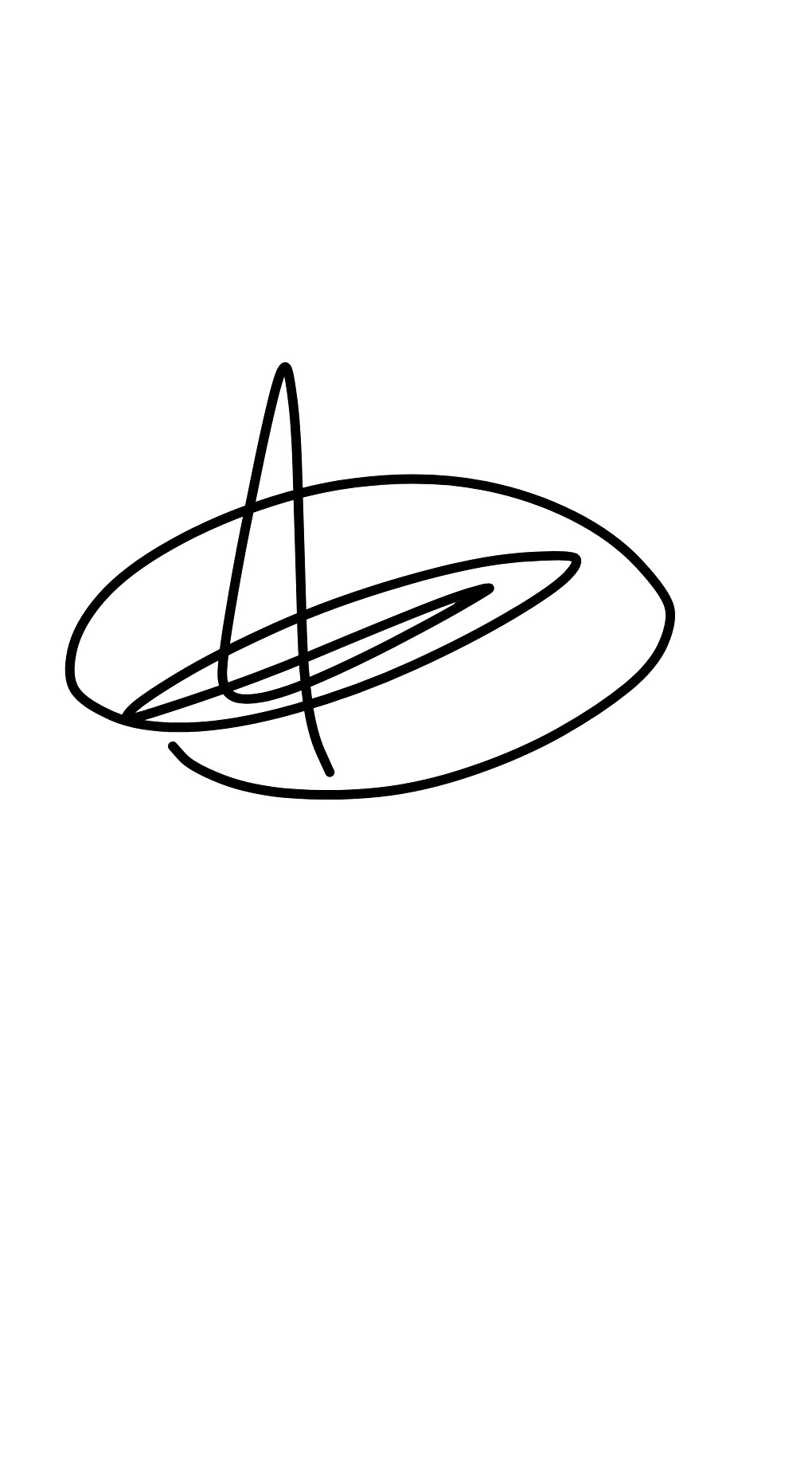On a completely white background, this image presents a black scribble that combines the erratic form of an illegible signature with the peculiar shape of a flattened witch's hat. The scribble begins at the bottom left and forms a spiral pattern, creating two concentric ovals, each smaller than the last, nesting within one another. At the center of the smallest oval, a V-shaped spike emerges, reminiscent of a paperclip or a spiked triangle, adding a distinct focal point that juts slightly upward to the right. The overall impression is one of a whimsical, yet somewhat chaotic design, resembling both a mishandled signature and a stepped-on witch's hat with a slight forward tilt, topped off with the appearance of a black-trimmed edge.